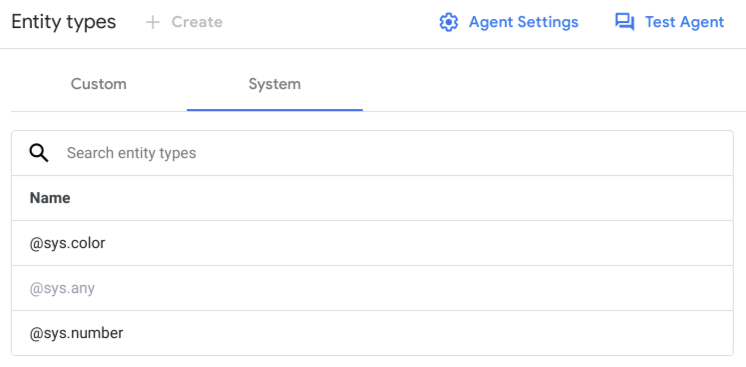The image appears to be a screenshot of either a web page or an app interface, likely associated with some kind of AI or chatbot management system. Here is a detailed and cleaned-up caption for the image:

---

The screenshot depicts a primarily white interface with black text, likely from a web page or app for managing AI agents. In the upper-left corner, there’s a section titled "Entity Types" in black text, accompanied by a grey plus sign labeled "Create." The upper-right corner features blue text next to a gear icon labeled "Agent Settings" and a small speech bubble icon labeled "Test Agent."

A thin grey horizontal line runs across the interface, beneath which are the words "Custom" and "System" in grey text. The word "System" is underlined in blue, indicating it is the selected option. Below this, a thin grey line extends horizontally.

The lower part of the interface contains a search box labeled "Search Entity Types" in grey text, with a small black search icon to its left. Below the search box, there's a section titled "Name" in bold black text. Under this section, "@sys.color" is listed in black text, followed by "@sys.any" in grey text, and "@sys.number" in black text at the very bottom right.

The overall design hints at a technical page dedicated to configuring or managing various entity types for an AI or chatbot agent.

---

This detailed description captures the key elements of the interface and provides context for its possible use.